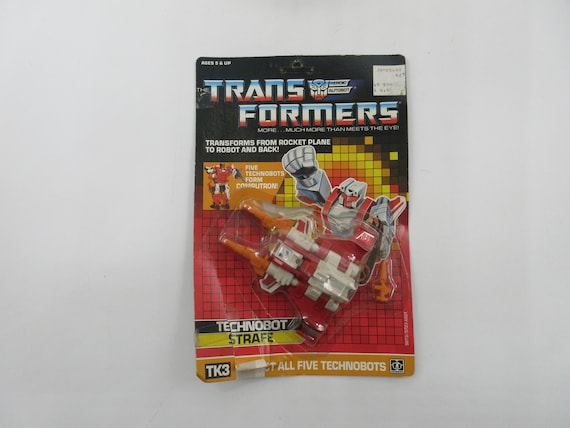In this horizontal rectangular image, set against a light gray background, a child's toy package is prominently displayed. The package features a Transformers toy encased in a combination of cardboard backing and a clear plastic bubble. The top third of the packaging displays a black heading with the word "Transformers" in bold letters, followed by smaller, less legible text. The lower portion of the packaging transitions into a yellowish and red background, housing the toy.

Inside the plastic bubble, several components of the toy can be seen. One figure appears ready for action, resembling a Transformer character with a fist prominently pumped out. Below this figure, there are two additional white plastic pieces that could be interpreted as ammunition or components that integrate with the Transformer figure. Above these pieces, there are drawings indicating the possible transformed states of the toy. The packaging also contains text mentioning "Technobot Strength" and "TK3," suggesting this toy is part of a series featuring all five Technobots.